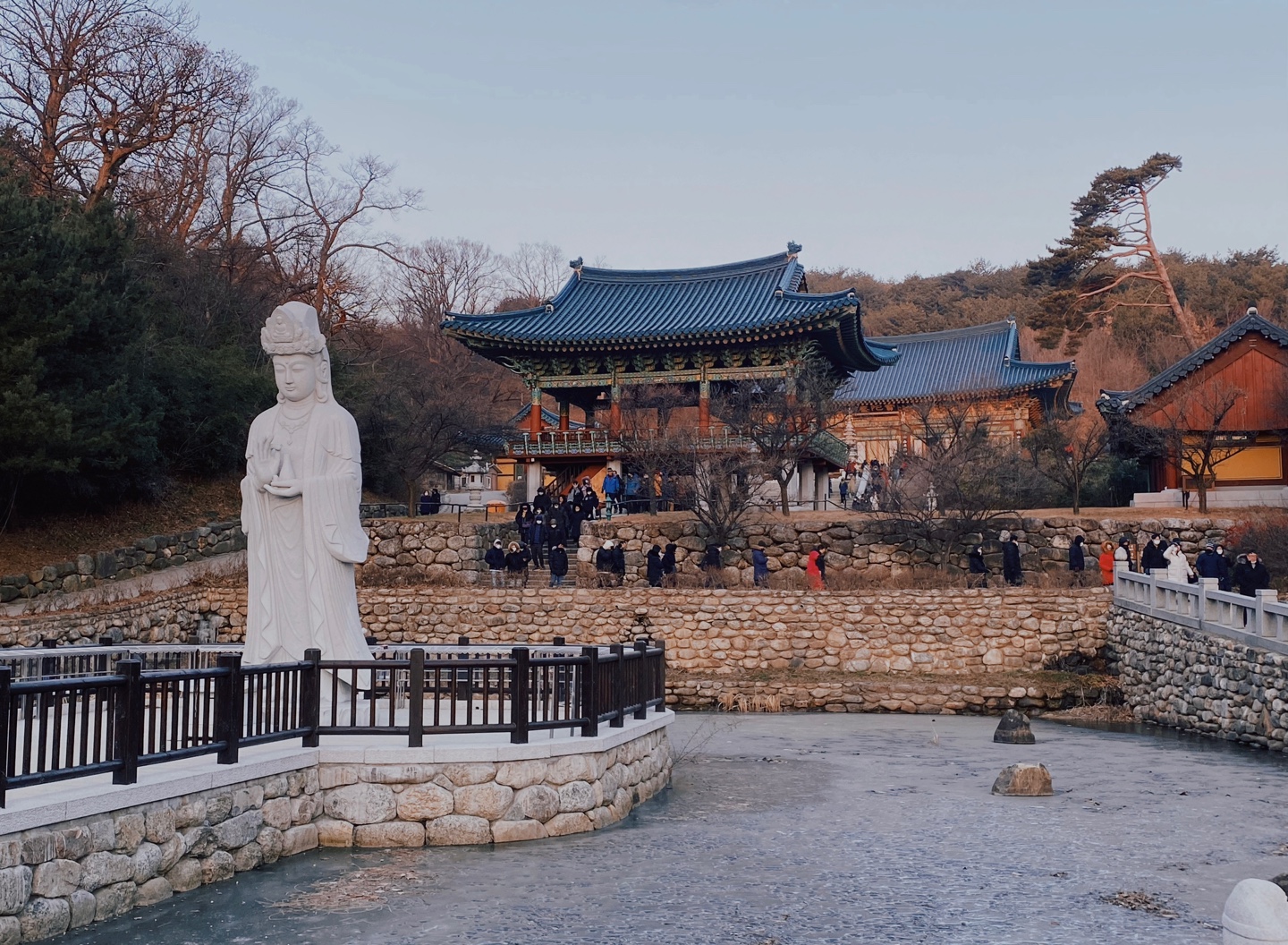In this daytime photograph, a traditional East Asian building, possibly Japanese or Chinese in architectural style, stands prominently against a clear blue sky. The building, featuring a distinct blue roof, is surrounded by numerous visitors exploring its grounds. Towards the upper left of the image, clusters of trees add a lush green background to the scene.

The foreground showcases a significant white stone statue of a woman, which stands on a platform within a body of water, suggesting a serene garden setting. This statue is encircled by a black wrought iron gate, adding to the structure's historical and aesthetic appeal. The location is paved with cobblestones and stone walkways, with a secondary stone structure that might serve as a bridge, enhancing the picturesque quality of the area. The combination of natural and architectural elements indicates a harmonious blend of cultural heritage and outdoor space, likely making this a popular tourist destination.